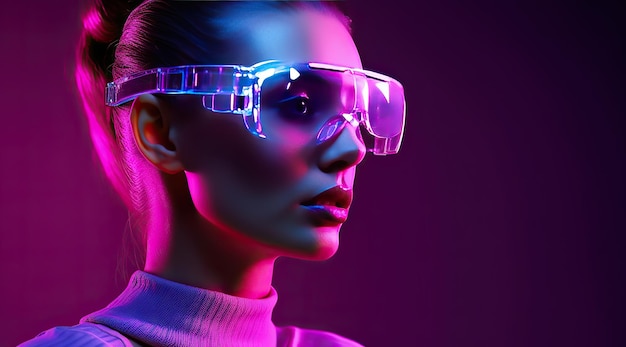This horizontally oriented photograph features the side profile of a young woman wearing clear, visor-style safety goggles that give off a futuristic vibe. Her hair is tied back in a ponytail, which complements the modern look of her transparent goggles, reflecting shades of pink and purple light. She’s dressed in a white turtleneck sweater, though the image cuts off just below the collar, leaving the full garment unseen. The lighting dramatically accentuates her face with a reddish illumination at the rear of her head, while the background is primarily dark, more lit on the left side and fading to black on the right. Her lips appear glossed, adding a subtle sheen that interacts with the ambient colors. This sophisticated, high-tech aesthetic suggests she might be a professional woman involved in a specialized or promotional context.